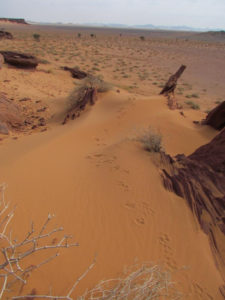In this blurry, yet intriguing desert scene, the image depicts a vast expanse of sandy terrain tinted with a light bronze or orange hue, evoking a surreal, Martian-like landscape. The foreground features a cluster of dried sticks and what appears to be a desiccated bush or tumbleweed, devoid of leaves. Scattered around this area are additional withered sticks and branches lying horizontally. The sand is marked with small animal tracks, indicating recent passage of a four-legged creature. Sparse, brushy foliage punctuates the barren wasteland that stretches across the scene. To the right, a stick juts out of the ground, and nearby, a modest hill rises from the desert floor. The distant horizon is outlined by a low mountain range, while to the left, a plateau of rock looms, adding to the rugged and inhospitable beauty of the landscape.